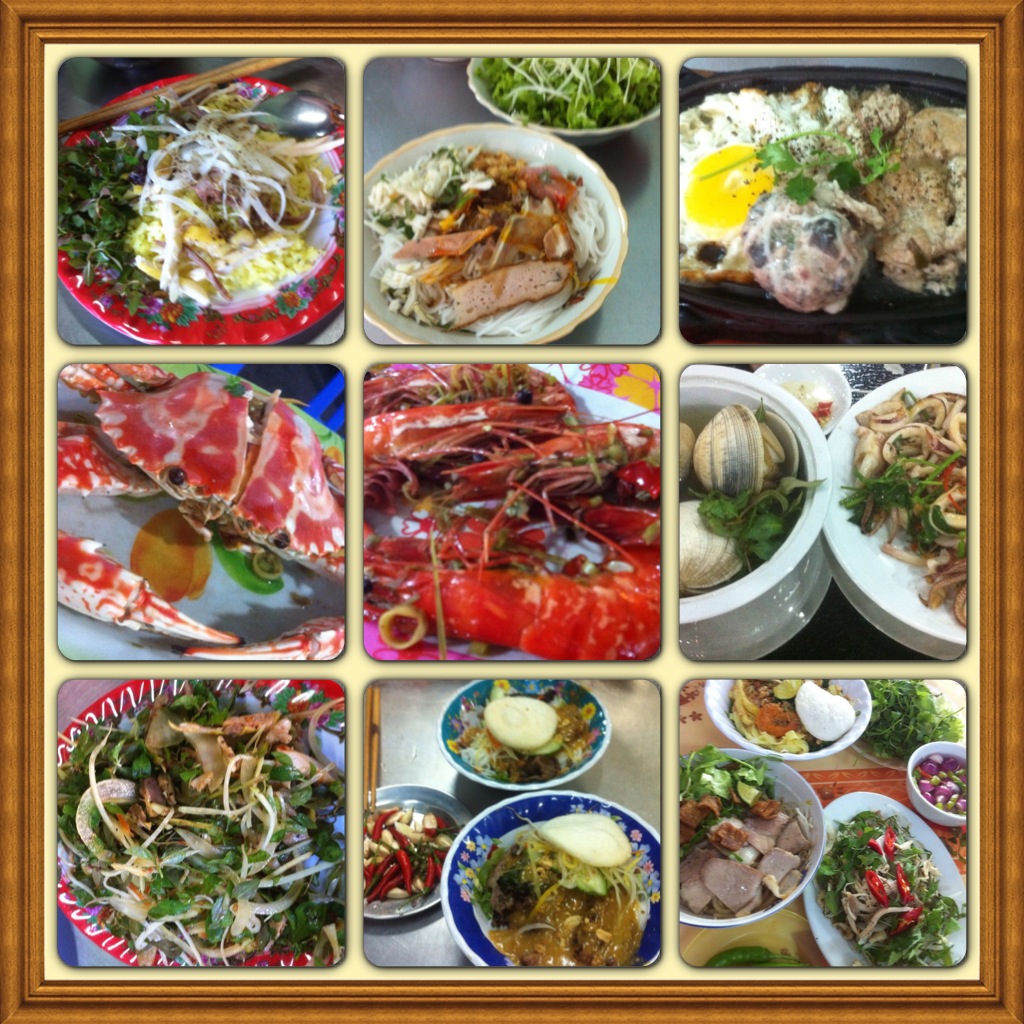A visually striking, square-shaped collage set within a light brown, indented frame displays nine distinct food images arranged in a tic-tac-toe format, with a soft yellow background peeking through the gaps. Each photo captures a seafood-themed or varied dish, served on intricately designed plates. In the top-left square, a vibrant red plate holds a dish featuring a yellow ingredient, presumably scrambled eggs, garnished with greenery. Moving clockwise, the top-center image showcases a round deli food item, flanked by noodles and a white bowl of salad. The top-right highlights a large fried egg on an unknown brown base. The center-left reveals a dead crab split open, while the middle houses a possible lobster or crab dish. The central-right depicts several red shrimp. The bottom-left square hints at shellfish, perhaps mussels, with one opened revealing its contents. Bottom-center and bottom-right photos feature various dishes, one including a bed of salad and another a collection with meat, bowls of soup, and salads, complete with colorful peppers. Despite the varied presentation, the shared repetition of seafood elements and vibrant reds across the dishes unify the collage.